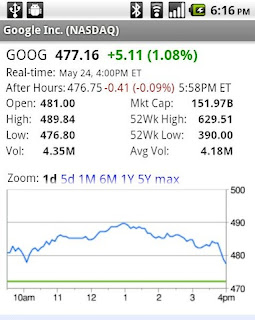This image captures a vintage user interface of Google Inc. stock information, likely from an early 2000s device, possibly a phone or iPod. The time displayed on the top right corner is 6:16 p.m., and it features early graphical elements typical of the period. The screen shows three white Wi-Fi bars within a black square icon, and next to it, a Bluetooth icon in another black square. 

Underneath, the screen lists the stock details for "Google Inc." with the NASDAQ symbol (GOOG). The displayed stock price is 477.16, with a green increment of +5.11 (1.08%). It notes the real-time update was at May 24th, 4 p.m. Eastern Time, and after-hours trading price at 476.75 with a red decrement of -0.41 (0.09%) at 5:58 p.m. Eastern Time.

Additional details include the day's stock opening at 481, the high at 489.84, the low at 476.80, a volume (VOL) of 4.35 million, and a market capitalization (MKT cap) of 151.97 billion. The 52-week high was 629.51 and the 52-week low was 390, with an average volume (VOL) of 4.18 million.

Below this data, the interface provides options for zooming into different timeframes: one day, five days, one month, six months, one year, five years, and maximum period. The "one day" option is highlighted in bold black, while the others are in blue. The graph underneath shows stock fluctuations between 470 and 490, with a horizontal green line indicating the time range from 10 a.m. to 4 p.m.